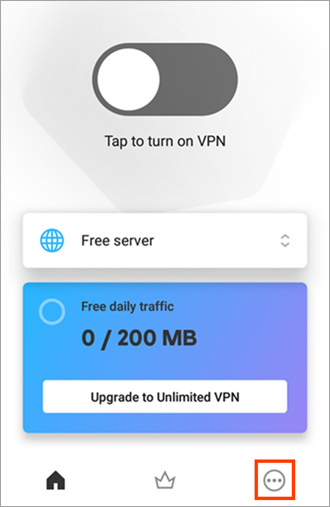The image appears to be a screenshot from a cell phone, depicting a VPN application interface. The background of the interface features a light bluish tone at the top. A large slider control, consisting of a white circle on a gray bar, is positioned to the left. Above the slider, black text reads, "Turn on VPN."

Beneath this section, there is a rectangular button with a white background. To the left of this button is an icon of a bluish-gold globe. The text within the button, also in black, states, "Free Server."

Lower down, on a blue background, there is a circular area and it displays "Free Daily Traffic" in black text. It further specifies "0 / 200 MBs," indicating that the daily limit of 200 megabytes has not yet been consumed. 

Following this, another section with a blue and white background contains black text urging the user to "Upgrade to Unlimited VPN."

At the bottom of the screen, there are three icons arranged in a row. On the left is a black house icon, in the center is a gray crown icon, and on the right is a circle containing three gray dots. Encircling these icons is a square with a red border.

The screenshot captures the entirety of the app's main interface, awaiting user interaction.